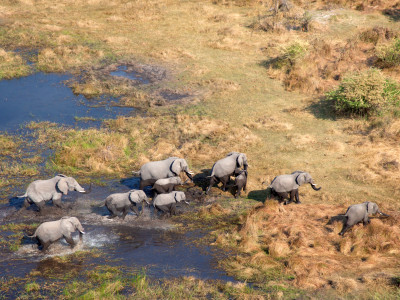In this captivating bird's eye view photograph, we observe a dynamic herd of elephants moving from water to land. The image is wide and vertically oriented, showcasing a sweeping landscape from a high vantage point. On the left side of the image, there are two circular, jagged-edged ponds or large puddles with shallow blue water. The surrounding land is a mosaic of different shades of brown, dotted with clumps of light and dark green grasses and shrubs.

The elephants, magnificent large creatures with their familiar gray skin, long trunks, and substantial ears, are either stepping out of the water or making their way towards dry ground. Those emerging from the water appear darker brown where they are wet. Beginning at the bottom left, two elephants stand side by side in the water, followed by another pair just ahead. A line of four elephants extends from this group, curving down towards the bottom right of the image. The herd appears as a coherent unit, some already on the land and others about to leave the water. Their organized procession creates a visually striking pattern against the variegated backdrop of the terrain. The detailed texture of both the elephants and the landscape offers a rich, immersive glimpse into the natural movement and environment of these majestic animals.